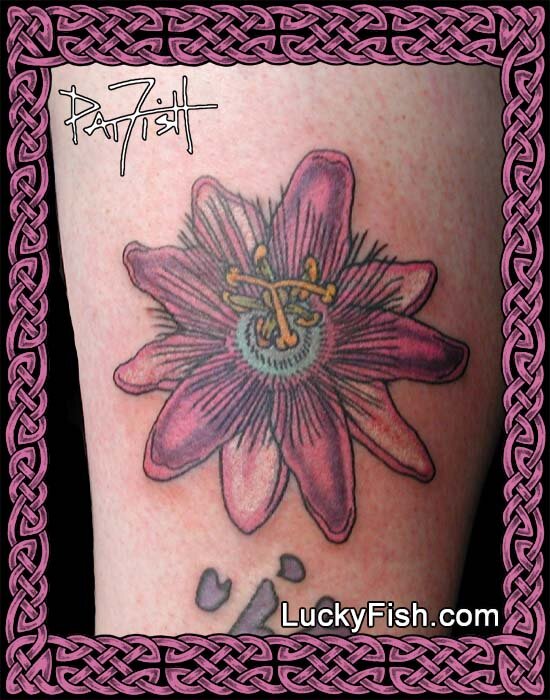In this detailed image, a section of a person's inner arm, right above the elbow, is adorned with a large, intricately designed tattoo of a pink flower. The flower boasts 13 petals and measures approximately 3 inches in diameter. At its core, the flower features a distinctive blue, button-like center, surrounded by delicate, black wispy threads and small yellow pollen nodules. The individual's skin is white with subtle red splotches.

In the top right corner of the image, the name "Pat Fish" appears in white letters with black contours, likely referencing the tattoo artist. Additionally, the bottom right corner bears the URL "luckyfish.com," also in white. The photograph is framed with a decorative border resembling interwoven Celtic or Irish designs, incorporating purple braided leather-like ribbons against a black background. The arm also hints at another tattoo partially visible below the pink flower, though it remains obscured.